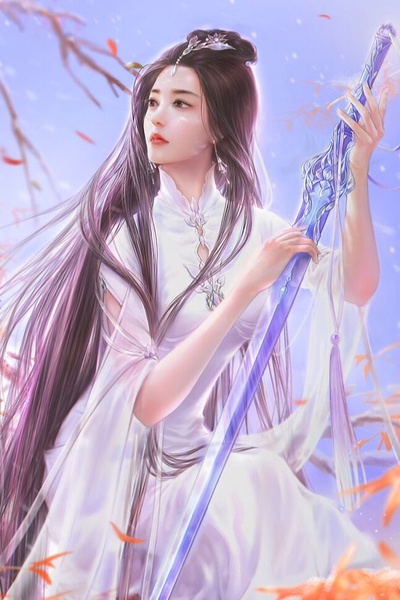In this detailed and artistically illustrated rectangular image, we see a beautiful young Asian woman with long, flowing black hair cascading past her waist. Her fair skin contrasts with her elaborate, white, chiffon-like gown, which features an Asian-style collar and a slight opening at the chest, revealing part of her fair skin. Adorned in long, dangly earrings and jewels that form a bead-like pattern across her forehead, she exudes a gentle yet captivating presence.

Her head is slightly tilted to the left as she gazes calmly to her right, displaying her small, arched eyebrows and a closed mouth. She holds a large, almost transparent blue crystal dagger, with hints of purple and lavender, adding an element of fantasy to the scene. Surrounding her are delicate branches, possibly cherry blossoms, along with vibrant orange and white flowers. The sky behind her is a light, periwinkle blue, casting a bright and serene light over the entire setting. The overall composition combines elements of fantasy and beauty, capturing both grace and strength in a striking visual.